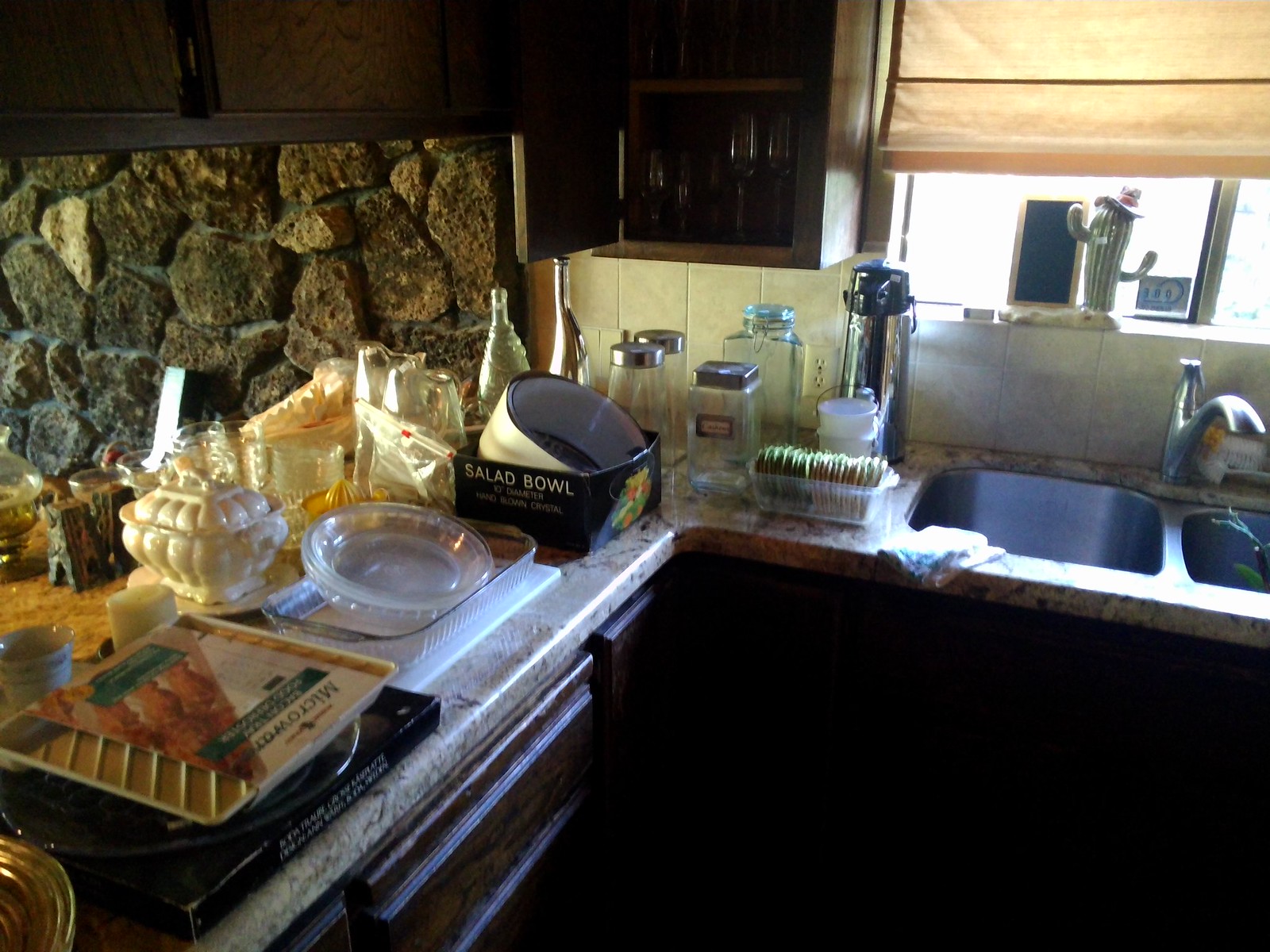A photograph showcases an L-shaped kitchen brimming with various cooking utensils, bowls, and other items scattered across the stone benchtop. The kitchen features a double sink positioned before a window adorned with Roman blinds, drawn halfway to let in natural light. Light peach-colored wall tiles cover one side of the kitchen, offering a warm and cozy ambiance. An opening from the kitchen leads to an outdoor area with a rustic stone wall in the background.

On the benchtop near the sink, a water thermos and several empty glass jars are neatly arranged. Adjacent to them are slender-necked glass bottles, adding a touch of elegance to the countertop. A salad bowl is placed inside a black box, accompanied by white ceramic pots with lids, likely used for storage. Additionally, there are a few round glass plates, and a dish rag is casually placed on the edge of the kitchen sink.

The kitchen's benchtop is made of a polished stone material, providing a sleek and durable surface for cooking and preparation. The cabinets, crafted from dark brown wood, offer a rich contrast to the lighter elements in the space, enhancing the overall aesthetic of this well-used and inviting kitchen.